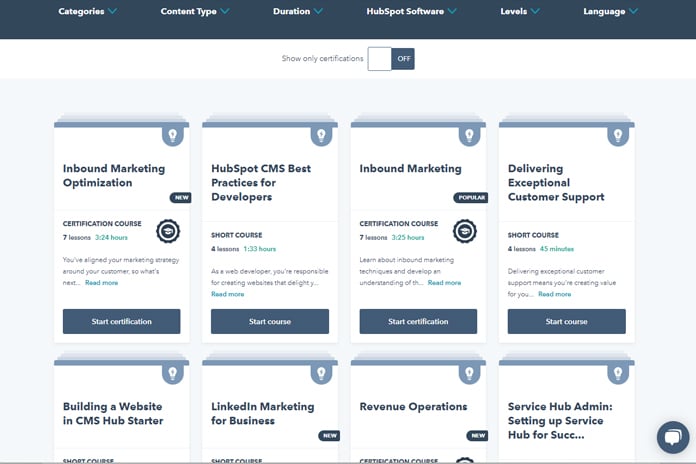This is a screenshot of an unidentified website showcasing various professional courses. At the top of the page, there is a sleek black banner with navigation options labeled Categories, Content Type, Duration, HubSpot Software, Levels, and Language. Below this, there is an option labeled "Show Only Certifications," which is toggled off.

The main content area is populated with several square tiles, each representing a different course available on the site. 

- The first tile is titled "Inbound Marketing Optimization" and is marked as 'New'. This is a Certification Course composed of 7 lessons, totaling 3 hours and 24 minutes. The brief description hints at advancing marketing strategies centered on customers. Options to "Read More" and "Start Certification" are provided.

- The second tile features "HubSpot CMS Best Practices for Developers." It's a Short Course that includes 4 lessons for a total of 1 hour and 33 minutes. The course is geared towards web developers with a focus on creating user-delightful websites. Options to "Read More" and "Start Course" are available.

- The third tile is labeled "Inbound Marketing" and is tagged as 'Popular'. It's another Certification Course, consisting of 7 lessons that span 3 hours and 25 minutes. This course aims to deepen understanding and techniques of inbound marketing. Again, options to "Read More" and "Start Certification" are offered.

- The fourth tile is titled "Delivering Exceptional Customer Support." It’s a Short Course with 4 lessons lasting 45 minutes in total. It focuses on creating value through exceptional customer support. Options include “Read More” and "Start Course."

Below these highlights, another row of course tiles is partially visible, featuring courses such as "Building a Website in CMS Hub Starter," "LinkedIn Marketing for Business," "Revenue Operations," "Service Hub Admin," and "Setting up Service Hub for Success."

The layout effectively presents a wide array of learning opportunities, categorized and detailed to facilitate user selection.